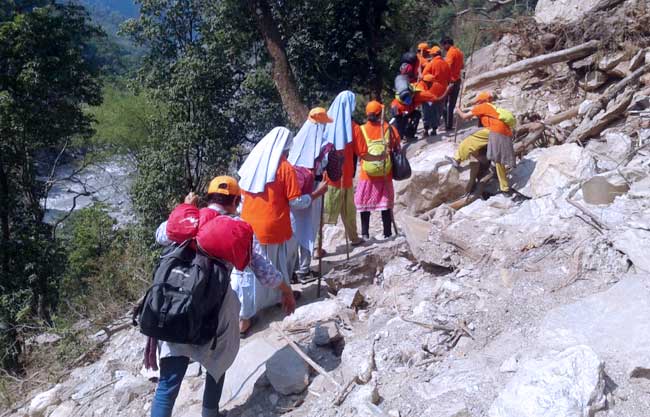The image depicts a group of approximately ten people, including both men and women, hiking up a steep, rugged, and rocky mountainside. The dominant color in the image is orange, as most of the hikers are wearing bright orange shirts. Additionally, many of the men are adorned with orange baseball caps, and one woman is also wearing an orange cap. Some of the women in the group have their heads covered with white veils or scarves, reminiscent of nuns' habits, although these veils appear simple and fabric-like rather than ornate.

The hikers are equipped with walking sticks and backpacks, suggesting the challenging nature of the terrain. They are ascending what seems to be a mountainous outcrop, navigating the difficult, loose rocks. The scene in the foreground highlights the rocky terrain, while the background offers glimpses of a possible river or rapids amidst trees and more rocky landscape. The photograph captures the backs of the hikers as they carefully traverse this demanding environment, emphasizing the arduous journey they are undertaking.